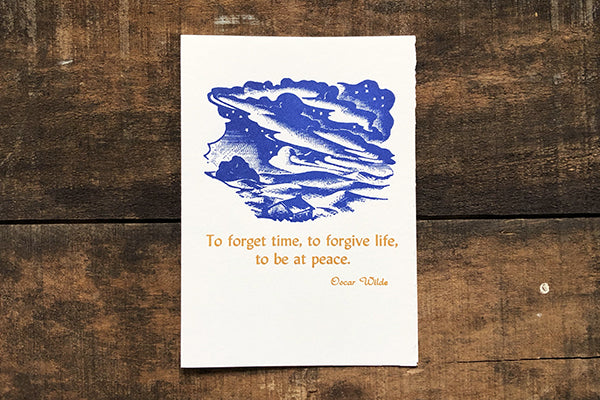In the center of this image is the cover of a white card. Prominently displayed in the middle of the card is a poetic line that reads, "To forget time, to forgive life, to be at peace." The quote is elegantly rendered in light golden font. Beneath this line, towards the right, is the name of the author, Oscar Wilde, also in the same golden hue. Above the text, there is an intricate, textured illustration featuring a blue and white sky with fluffy white clouds, and a house situated below. The card is set against a dark brown and black wooden surface that adds a rich contrast to its pristine white color.